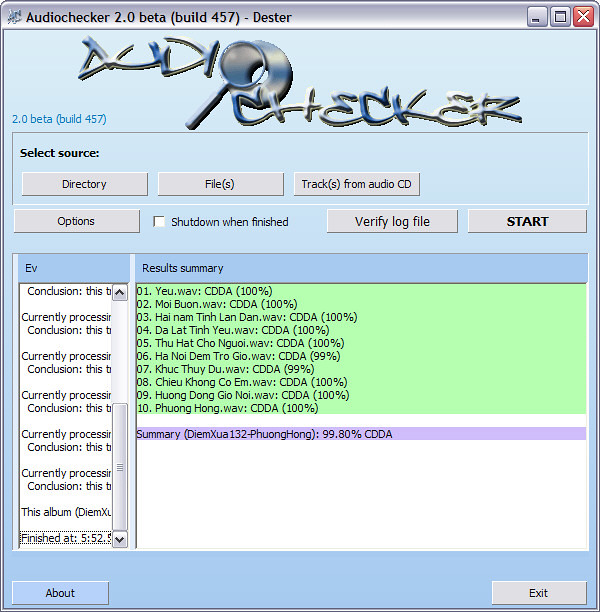The image shows a screenshot of the AudioChecker 2.0 beta (build 457 duster) software window, an older program designed for audio validation and analysis. The window's frame is light gray, with the program's name prominently displayed at the top. Just below, the stylized blue metallic AudioChecker logo features a magnifying glass between the words. Beneath this, blue text repeats "2.0 beta build 457," followed by black text reading "Select Source."

There are several gray buttons: "Directory," "Files," "Tracks from Audio CD," "Options," "Verify Log File," and a larger "Start" button. The main section, a white pane, displays a list of 10 tracks highlighted in green, each denoted as "0 1 YEU.WAV: CDDA 100%" indicating the file format and analysis results. The tracks, written in English letters but likely in Vietnamese, include titles such as "Moi Buon," "Hai Nam Ting Lan Dan," and "Da Lat Ting Yu," all in WAV format with a "CDDA 100%" accuracy rating. Additional purple-highlighted summary details specify detailed percentages for other tracks still being processed.

Icons in the top-right corner allow minimizing, maximizing, and closing the window. At the bottom of the window, there is a button labeled "About" on the lower left, and an "Exit" button in gray on the lower right. The overall aesthetic suggests the software dates back to the early 2000s, reflecting its vintage interface design.